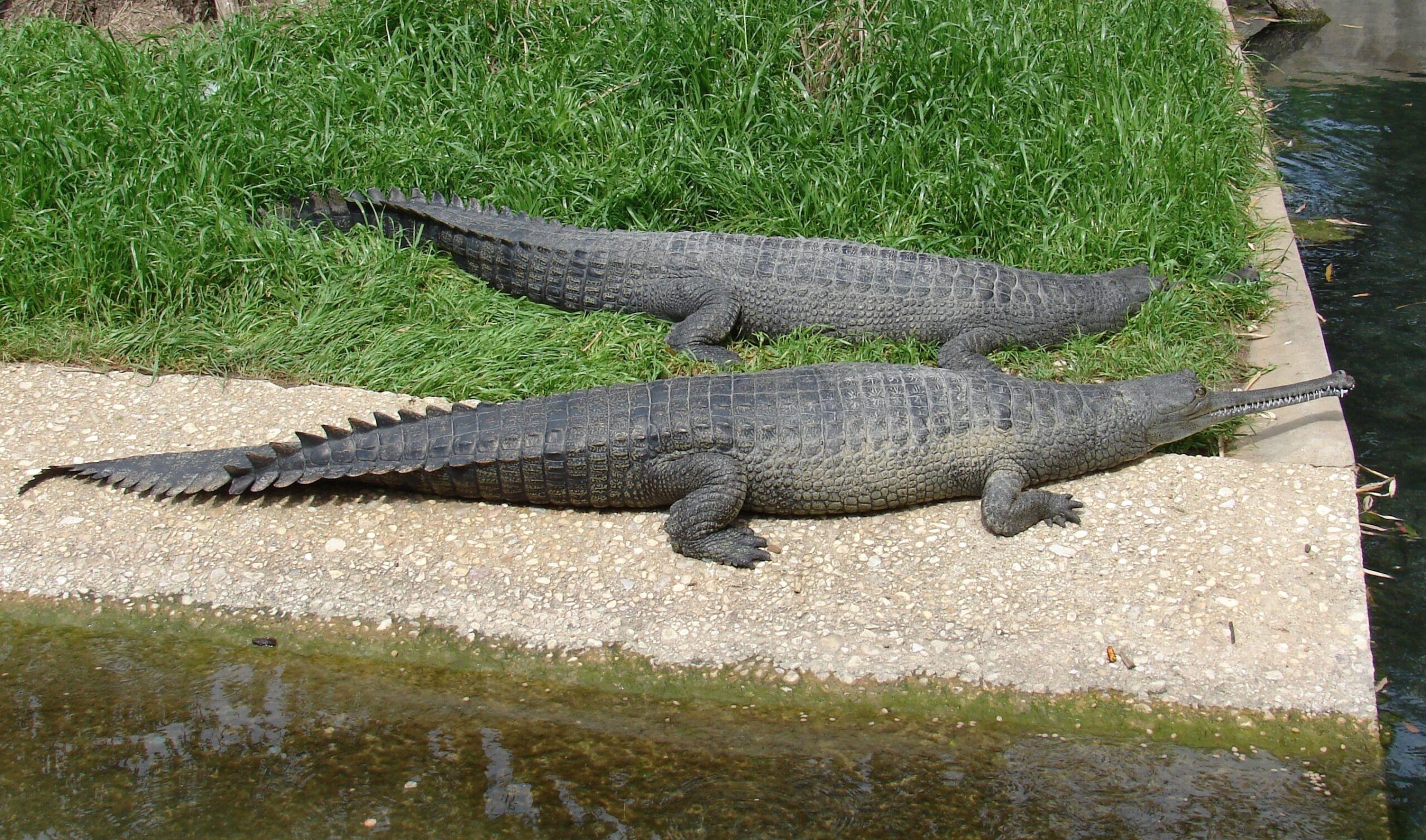The image depicts two crocodile-like reptiles basking on a concrete bank beside a body of water. Both have long, thin snouts filled with sharp, needle-like teeth and scaly, grayish skin. The larger of the two is sprawled mainly on a rough, light-brown concrete barrier that separates the water from the grass. Its tail almost reaches the left edge of the image, while the head is near the right. Spiky ridges run along its back, and its legs are curled under its body as it rests. The smaller reptile is positioned in the grass, partially obscured by the long green blades. Between the two, the grass appears flattened, contrasting with the taller growth behind them. The water, dark green with floating grass, is visible in the upper right section and lower right-hand corner, where it meets the mossy base of the concrete wall. The overall scene highlights the textured landscape and the distinct features of these peculiar crocodilian creatures.